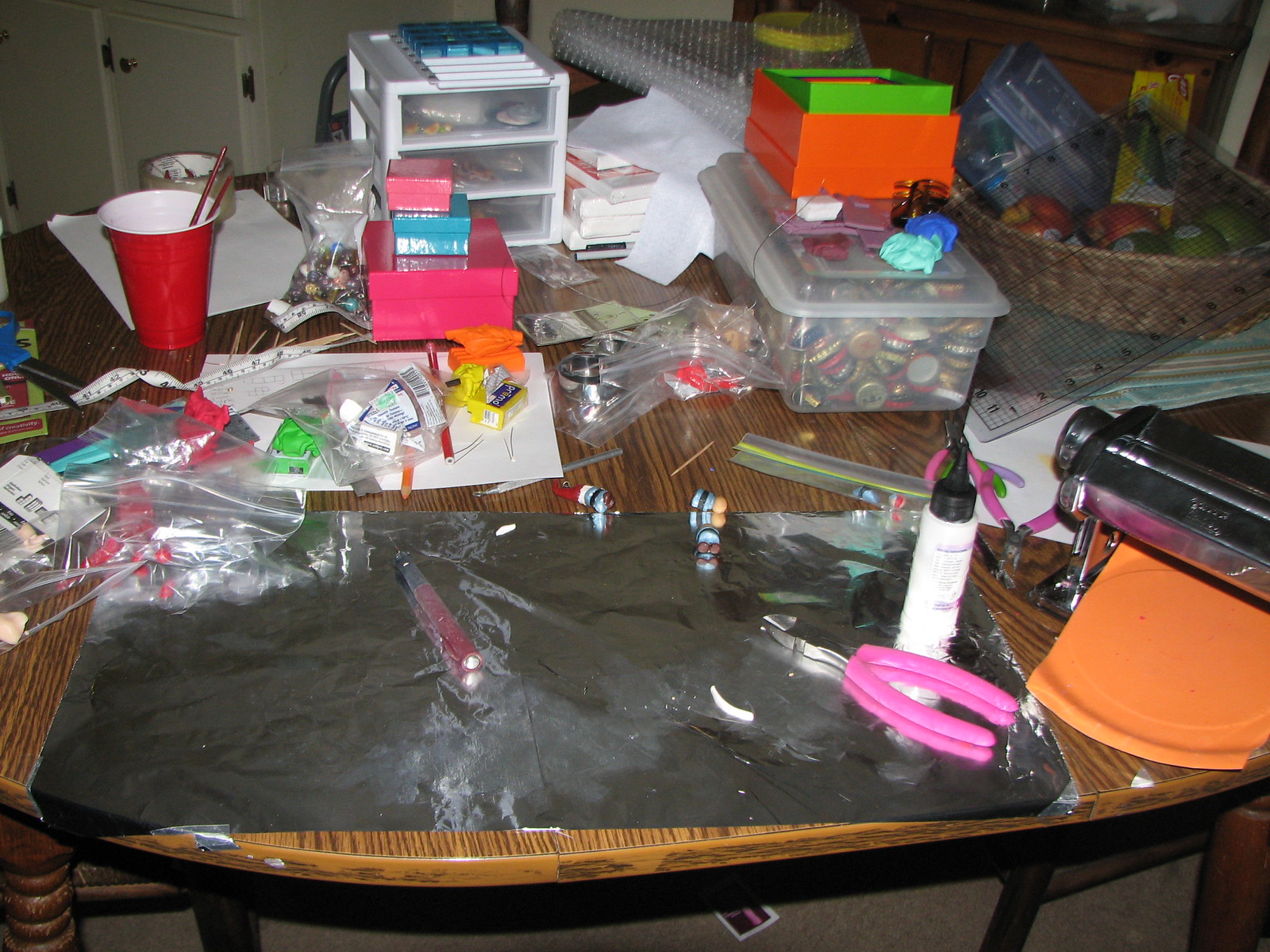This photograph captures a cluttered crafting table set against a brown wooden surface with matching legs extending to a brown carpeted floor. The table is strewn with various craft supplies. Dominating the foreground is a piece of foil taped to the table, holding a pair of pink pliers and a white bottle with a black lid. To the right of this setup lies a broken paper plate with a metal object resting on it. At the top right of the image, there is a brown basket filled with a variety of apples—green, red, and yellow. Adjacent to the basket is a yellow box.

Moving left from the yellow box, a clear container houses an assortment of beer bottle caps. Further to the left, several plastic baggies containing unknown items are scattered around. Near these baggies, a small pink box is stacked atop a blue one. Continuing with the organizational chaos, there is a clear drawer unit, a separate small baggie filled with buttons, and a red Solo cup holding paintbrushes. Finally, the table also contains a white piece of paper and a roll of tape, adding to the overall sense of disarray.